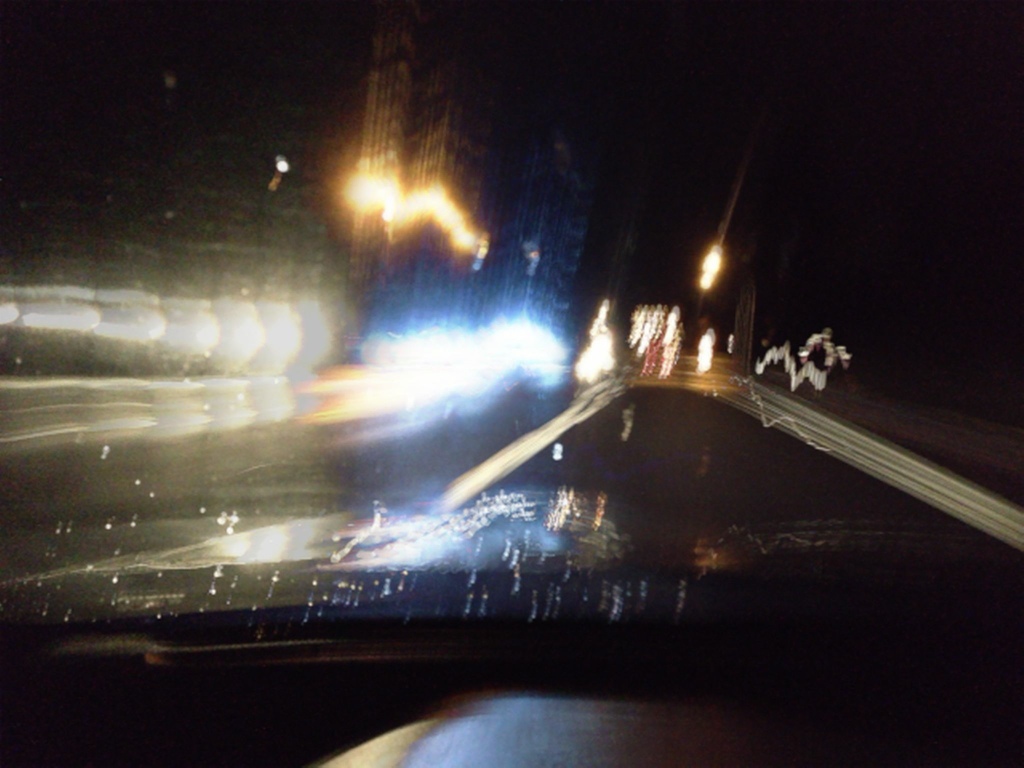A blurry nighttime photograph depicting an outdoor scene. The image features several indistinct street lamps casting a diffused glow, illuminating curved roads. Prominently, a winding road curves extensively on the right-hand side, where faint, white, elongated figures—possibly people—are visible atop the curve. The left-hand side showcases streaks of light radiating outward from the center, perhaps from passing vehicles or light reflections. At the bottom of the image, the presence of subtle, scattered remnants suggests recent rainfall, adding a reflective sheen to the scene.